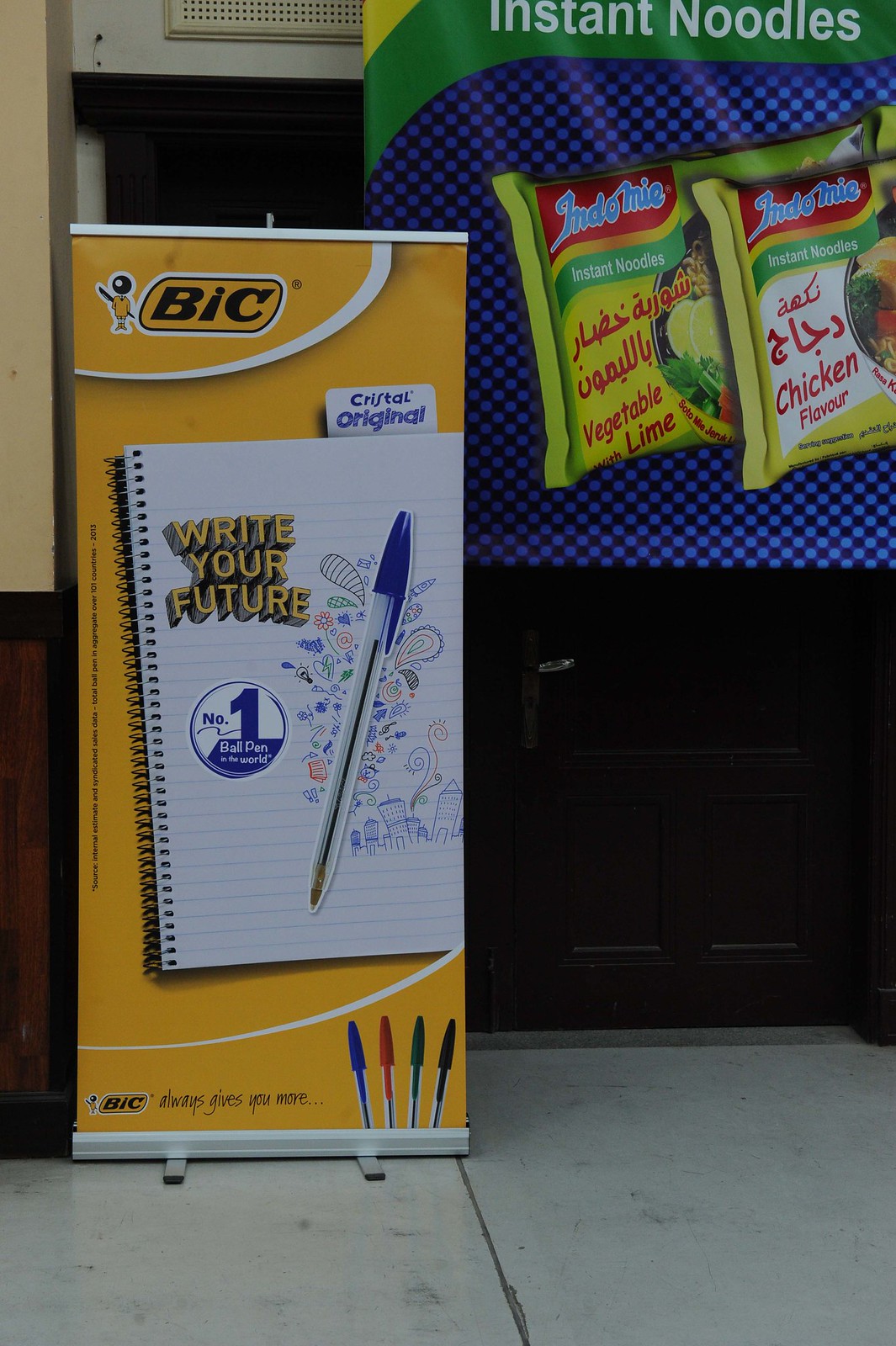In this image, we see a freestanding, tall advertisement poster situated on the left side, placed on the ground and supported by a metal stand. The poster features a vibrant yellow background. The prominent BIC logo, comprising the company name in black letters adjacent to a yellow oval containing a small animated character with a black ballpoint pen head, adorns the top left corner. Below the logo, the text "Write Your Future" is emblazoned on a large picture of a notebook, presented in an imitation pencil drawing style. Accompanying this is a blue circle with the words "Number One Ball Pen in the World." A clear blue-capped BIC ballpoint pen with scribbles and doodles in various colors surrounds the central image, adding a playful element. Towards the bottom of the poster, another tagline reads "BIC Always Gives You More," accompanied by images of four pens with differently colored caps (blue, red, green, and black).

On the right side of the image, a dark brown door is visible, above which another poster is attached. This secondary advertisement has a blue background with a green-yellow stripe and showcases packets of Indomie instant noodles in vegetable lime and chicken flavors, arranged against a black and blue checkered pattern. The setting is characterized by a light gray floor, suggesting the image was taken in a room possibly near an entryway.